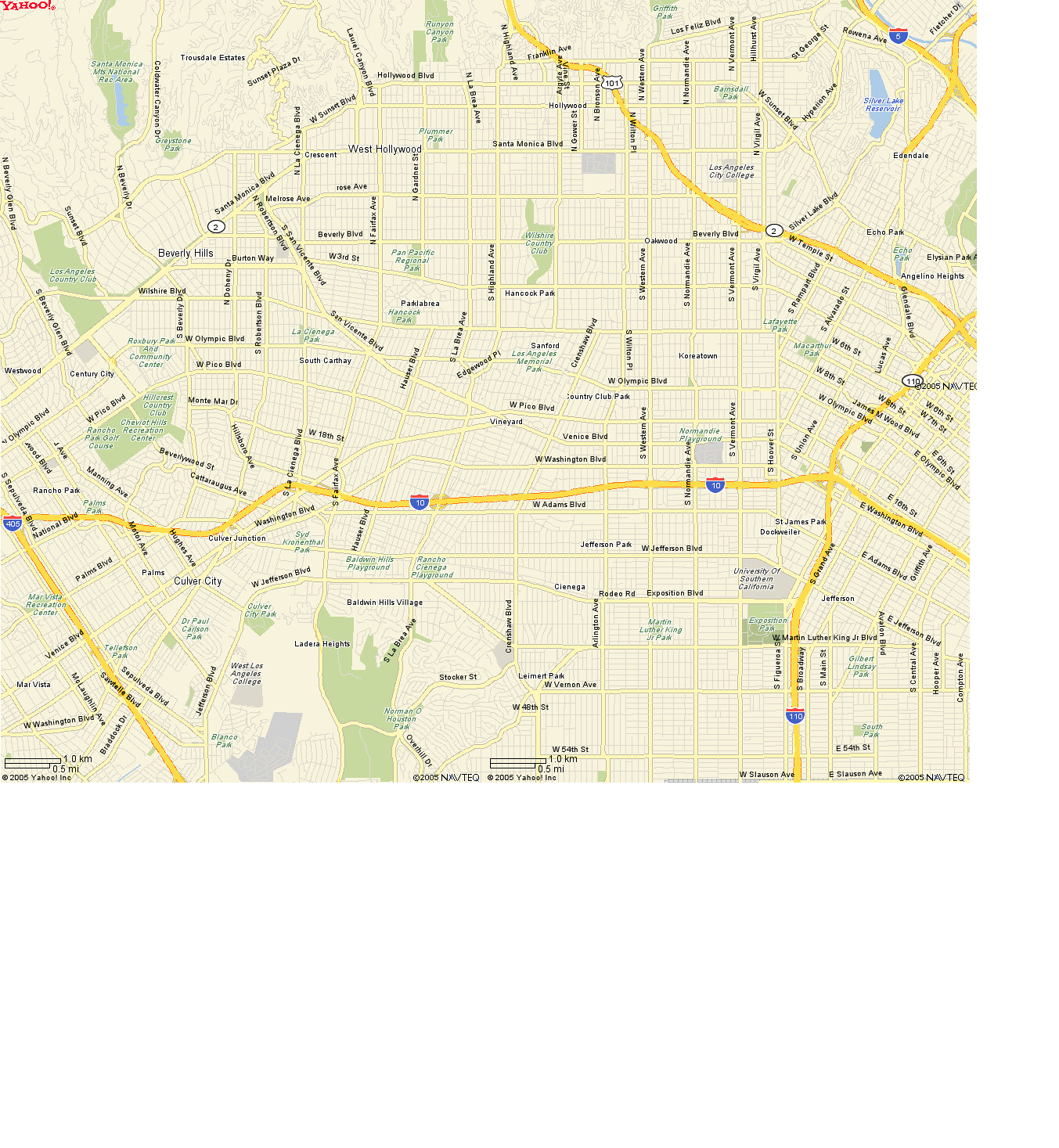This image depicts a classic map, likely sourced from Yahoo Maps, showcasing a detailed urban layout. Vertical and horizontal lines crisscross the map, representing a network of streets marked with tiny, black text indicating their names. Prominent on the map are bright yellow lines signifying various freeways and highways, which snake through the map with a distinctive curvature, particularly concentrated in the right section of the image. These highways feature special symbols resembling little shields, colored blue and red, denoting important routes. At the bottom, the map includes a mile or distance indicator, with identical bars and descriptions located in both the bottom-right and bottom-left corners. In the top-left corner, the word "Yahoo" is displayed in red text, hinting at the map's antiquity. Additionally, the map features blue shapes representing bodies of water and green areas indicating parks, adding to the overall complexity and richness of the urban landscape depicted.